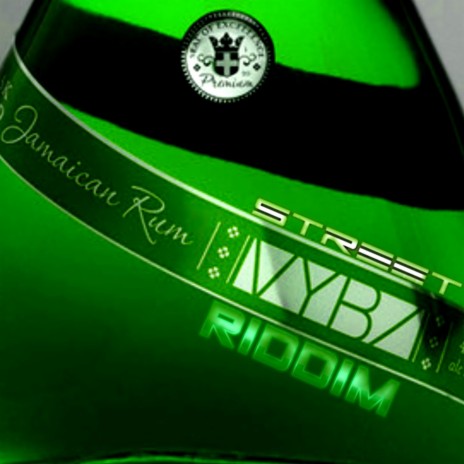The image is an extremely close-up view of a green bottle, presumably a bottle of Jamaican rum. The bottle occupies almost the entire frame of the image, with only slight portions of the grey background visible in the top left and right corners. The focal point of the image captures the upper section of the bottle, specifically near the neck where it transitions to the stem. 

A prominent seal is located at the upper part of the bottle. This seal is white with a detailed coat of arms, featuring a black shield and a grey cross. Below the seal, a green ribbon with white lettering wraps around the bottle. The text on the ribbon reads "Jamaican Rum" followed by "Street VYBZ Rhythm." The label appears to angle slightly from the upper left side of the bottle towards the lower right side. The overall scene emphasizes the intricate details and labeling of the bottle, highlighting its distinctive green color similar to that of a Heineken bottle.